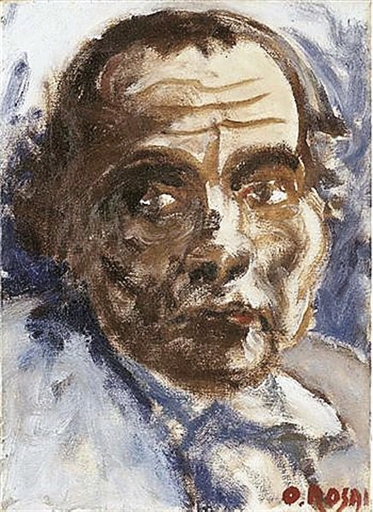This image is a color painting depicting a man's portrait executed in a loose, impressionist style with broad, rough brush strokes. The man's face, created with brown tones, appears somewhat dirty and blotchy, devoid of clear, definitive lines except for the forehead, which features casually painted wrinkles. His thick brown eyebrows and brown pupils, which look to the left, are more defined against the blurred, brown strokes that form the rest of his face and hair. The man has thinning, balding hair with a widow's peak, and he shows a mild grunt or frown on his jowly face. He is dressed in a white garment with a collar that protrudes in front of his chin, possibly a blue or white jacket. The background transitions from blue at the bottom to an off-white at the top, contributing to the impressionistic feel. Additionally, there is red writing at the bottom right corner of the painting that reads "O. Rosa," which might be an artist's mark or part of the artwork itself. The entire piece captures the essence of the subject with an artistic texture that emphasizes the paint's application on the canvas.